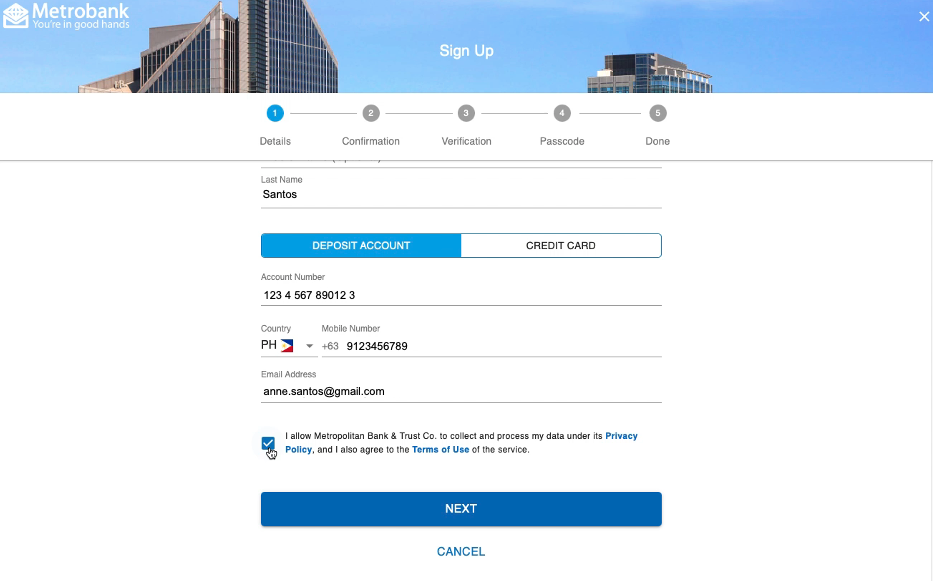The image depicts the Metrobank website interface. In the upper left corner, the recognizable Metrobank logo is displayed alongside the tagline "You're In Good Hands," both in white font. This heading is part of a banner stretching across the top of the image, framed by the blue sky, and positioned between two buildings which are separated by some space, allowing more blue sky to be visible.

Below the banner, the page appears to be a registration or sign-up form. The title "Sign Up" is prominently featured, followed by a progress bar indicating that the current step is "Details." Under this section, there is an input box pre-filled with the last name "Santos." Below the last name input, there are two account type options: "Deposit Account" and "Credit Card." The "Deposit Account" option is selected, revealing fields for "Account Number" and "Mobile Number" underneath.